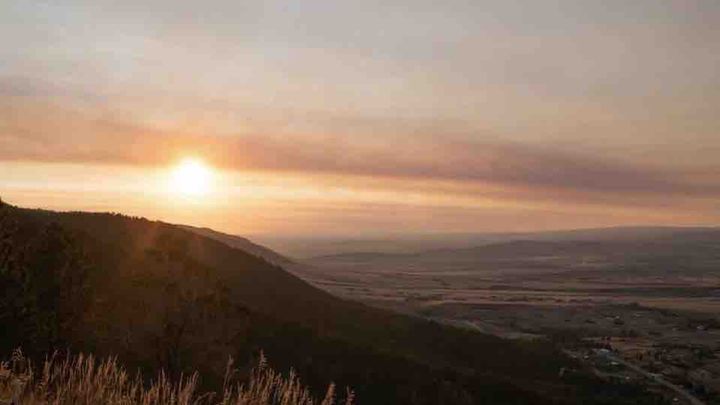This vivid color photograph captures a breathtaking sunrise over a sprawling landscape. Dominated by warm hues of orange and yellow, the sun is positioned towards the left side of the image, ascending above the horizon and casting radiant streaks of varying shades of orange across the sky. The foreground features a hillside covered with grassy plains and tall wheat, accentuated by tumbleweeds in the lower left corner. Below this hill, the land unfolds into lighter brown terrain, creating a layered visual effect that indicates the hill's elevation above the surrounding land. 

In the distance, the horizon reveals another smaller, darker brown mountain, adding depth to the scene. Despite the vintage, somewhat pixelated quality of the photo, one can make out a couple of houses nestled amidst the grassy expanse on the lower right corner, suggesting human presence. The near-cloudless sky, marked only by a single large cloud, reflects the sun’s rays, enhancing the photo's serene and timeless appeal.